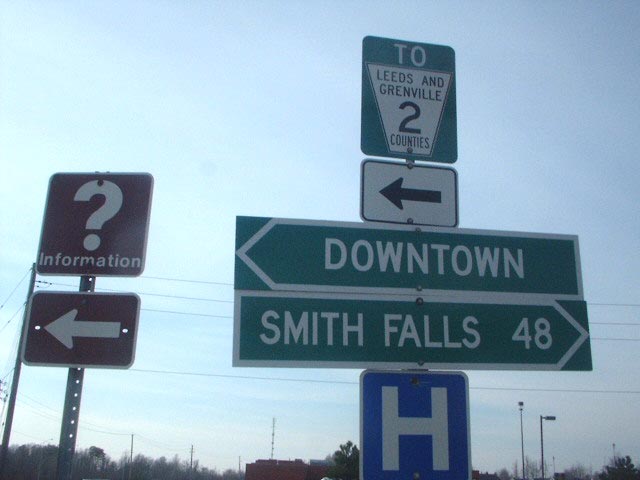The photograph features an array of road signs against a bright, glary light blue sky, free of visible clouds. Framed by a backdrop that includes the tops of trees, buildings, tall street lamps, and cell phone towers, the image captures a vertical stack of road signs prominently in the foreground on the right-hand side. At the top of this stack is an inverted triangle sign that reads "TO Leeds and Greenville, two counties." Below this is a rectangular white sign with a black arrow pointing left. Beneath that are two long, green rectangular signs with white lettering; the top one points left and reads "Downtown," while the bottom one points right and is labeled "Smith Falls 48." Underneath these is a blue square sign featuring a white letter "H" for hospital. To the left of this main stack is another metal pole bearing two brown signs. The top brown sign features a white question mark and the word "Information." Directly below it is another brown sign with a white arrow pointing left. The bright sky adds a bit of glare, making the signs stand out sharply as they guide travelers.